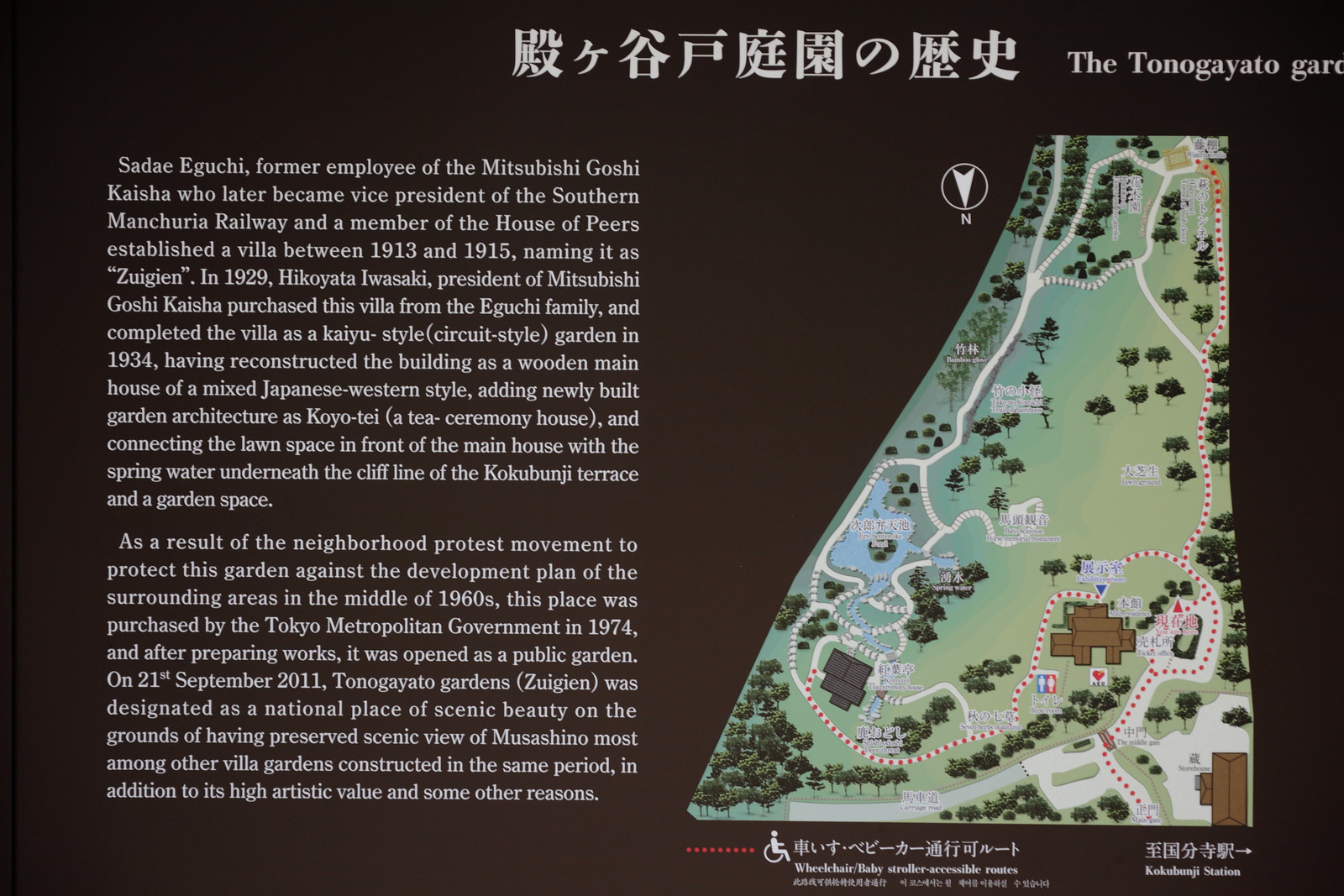The image is a photograph of an informational sign, likely found at the entrance or visitor center of a park, specifically the Tono-Gayato Garden. The sign has a black background with white text and is divided into two sections. On the right side, there is a detailed illustrator's map of the garden, showing paths, trees, bodies of water, houses, and bathroom spots. The map includes labels in Japanese and an arrow in the top corner pointing downwards with a capital 'N', indicating north.

At the very top of the sign, it reads "Tono-Gayato Garden" in English, accompanied by Japanese text. Below this title, the left-hand side of the sign contains two paragraphs of historical information detailing the garden's origins and development.

The text states that Sadie Eguchi, a former employee of Mitsubishi Goshi Kaisha who later became the vice president of the Southern Manchuria Railway and a member of the House of Peers, established a villa between 1913 and 1915, naming it Zuigien. In 1929, Hikeyota Iwasaki, president of Mitsubishi Goshi Kaisha, purchased the villa from the Eguchi family and completed it as a caillou-style circuit garden in 1934. He reconstructed the building into a wooden main house of mixed Japanese-Western style, added new garden architecture, including a tea ceremony house called Koyotei, and connected the lawn space in front of the main house with the spring water underneath the cliff line of Koku Bunji Terrace.

The sign also notes that due to a neighborhood protest movement in the 1960s against the development plans for the surrounding area, the Tokyo Metropolitan Government purchased the garden in 1974. After preparations, it was opened to the public on September 21, 2011. The Tono-Gayato Garden, also known as Zuigien, was designated as a National Place of Scenic Beauty because of its high artistic value and its preserved scenic views of Musashino, surpassing many other villa gardens from the same period. 

Lastly, the sign contains some Japanese text, a wheelchair icon, red dotted lines, and annotations marking the garden's various features.